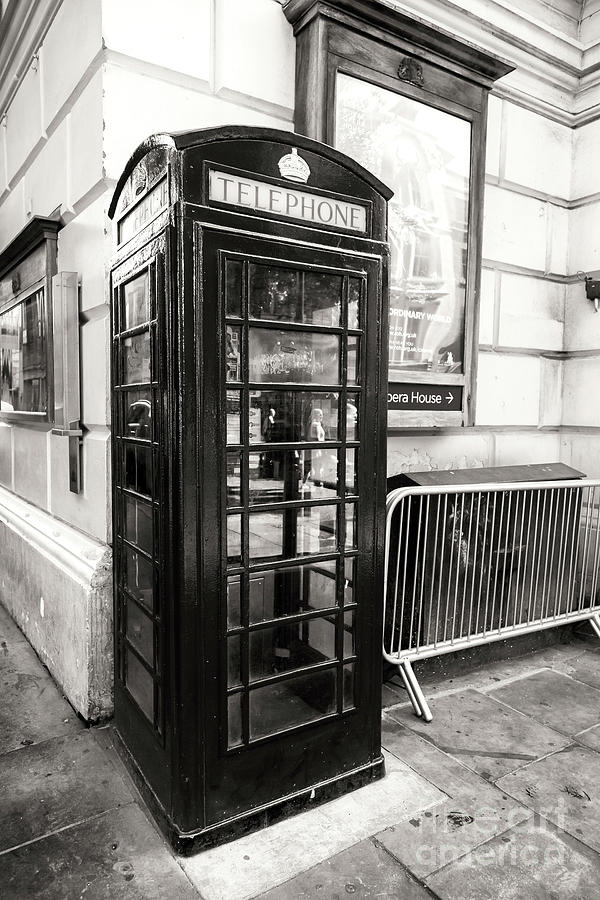The image is a black-and-white photograph capturing an outdoor scene at the corner of a brick building, likely from Britain. Central to the image is an old-style London telephone booth, characterized by its wooden structure, glass panels on all sides, and a "Telephone" sign at the top with a royal crown emblem above it. The booth, slightly worn with chipping paint, houses a payphone inside. To the right of the telephone booth, a metal barricade or fence is visible, possibly a barrier control. Behind the telephone booth, attached to the building, is a sign that reads "Opera House" with an arrow pointing to the right. The ground is made of stone bricks or old-style tiles, contributing to the historical ambiance of the scene. Another indistinct sign is on the left side of the wall, beyond a telephone pole. The overall atmosphere of the photograph evokes a sense of historic Britain.